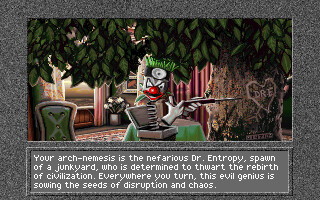This is a low-quality screenshot of what appears to be a video game, possibly a mobile game. The main focus is an ominous clown character emerging from a jack-in-the-box. The clown, distinguishable by its red nose, green hair, and headband with a white circle, has a coiled metal spring neck and is holding a sharp object that resembles a gun or a knife. It is insidiously carving the letters "DRE" into a tree trunk, where a heart with an arrow is etched. Surrounding the clown, the scene includes green chairs, a table, and foliage with leaves cascading down, suggesting an indoor environment possibly looking out to a skyline. Text appearing in a large box at the bottom reads, "Your arch-nemesis is the nefarious Dr. Entropy, spawn of the junkyard who is determined to thwart the rebirth of civilization. Everywhere you turn this evil genius is sowing the seeds of disruption and chaos." The image is bordered by a gray frame speckled with white, reminiscent of static on an old television screen.